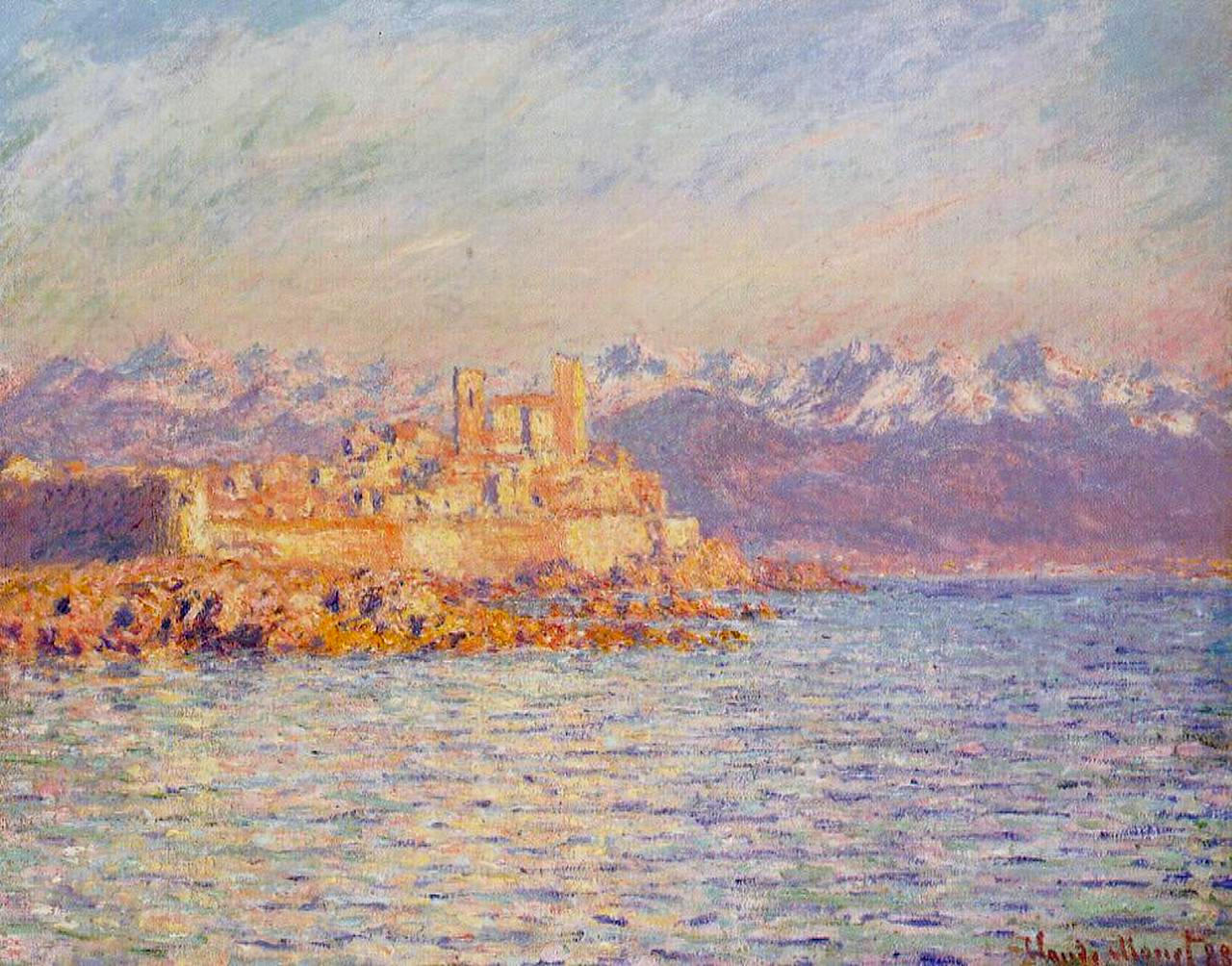This watercolor painting, attributed to Monet, captures a dramatic coastal scene. The central focus is an old castle positioned on an elevated clay city, with golden brown and beige hues illuminating its structures. The city, which includes various houses and buildings, is set against a vast, mountainous backdrop stretching across the width of the painting. The mountains begin rocky and transition to snow-capped peaks under a blue sky. In the foreground, small and large rocks dot the shoreline leading up to the blue and white sea. The waters and sky convey a mood that is neither tranquil nor turbulent, striking a balance between calm and unrest. The painting, wider than it is tall, is meticulously detailed with pronounced brush strokes and dramatic shading. The artist's signature, rendered in red paint, graces the lower right corner, confirming its creation by Monet.